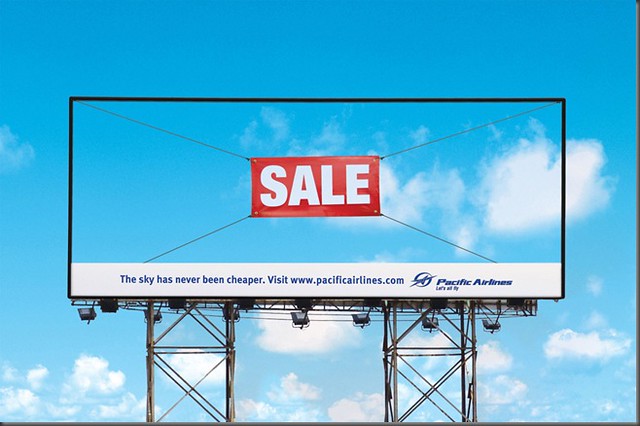The image captures a uniquely designed billboard advertising Pacific Airlines. The billboard features a captivating aesthetic with a hollow black frame that allows the actual blue sky with white clouds to be visible through it, blending seamlessly with the background. Suspended from each corner by black cables, a large red sign with "SALE" written in white text commands attention at the center of the billboard. Below this, a white stripe reads, "The sky has never been cheaper. Visit www.pacificairlines.com," followed by the Pacific Airlines logo on the bottom right. The billboard is mounted on a brown or copper-colored metal structure with lights at the bottom, enhancing its visibility and modern appeal. This clever design visually reinforces the advertisement's message by making the sky appear as if it's truly on sale.